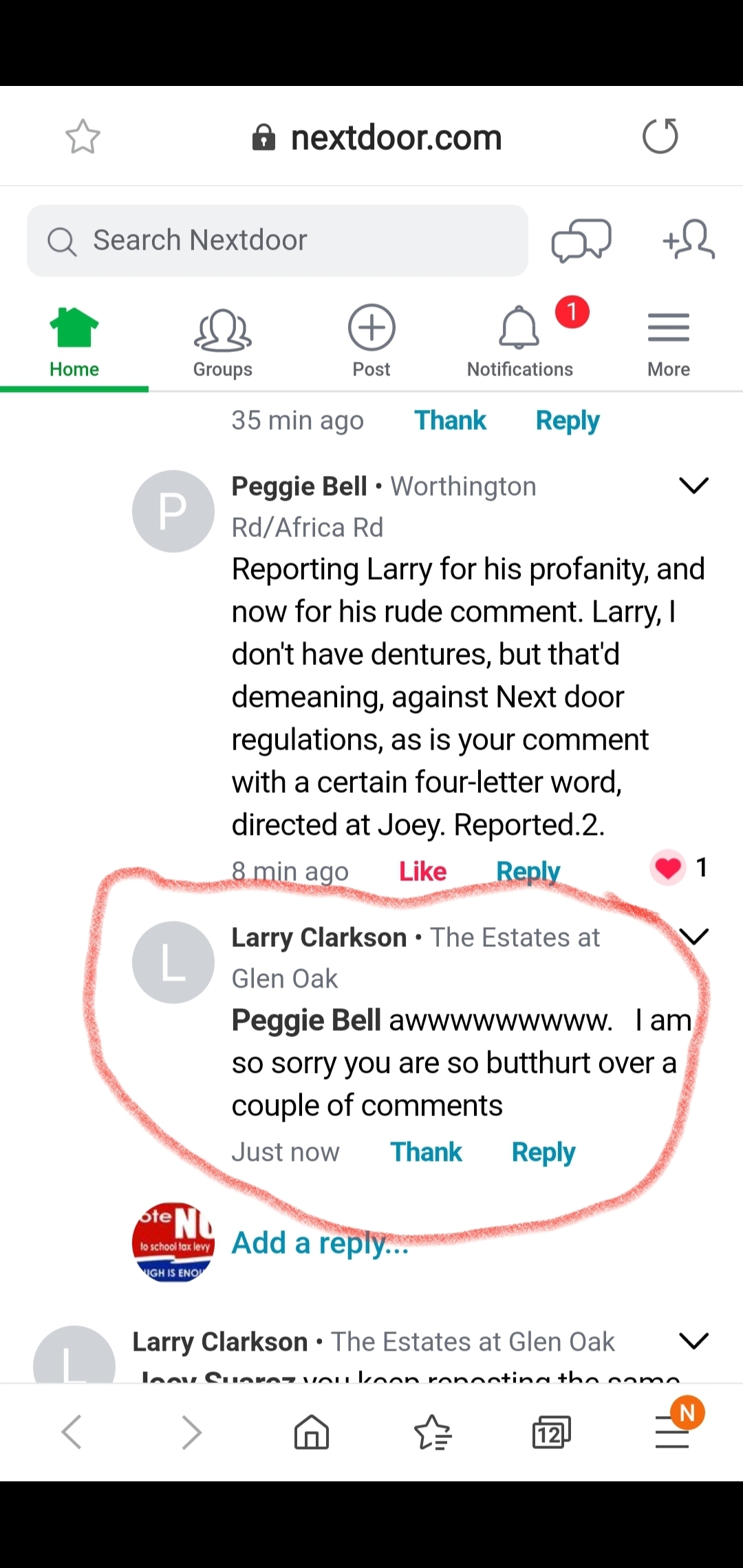This image appears to be a screenshot taken on someone's phone, displaying an interface from the Nextdoor app. At the very top of the screen, there is a black bar. Below this, the main interface features a white background. Prominently displayed is a black padlock icon accompanied by the text "nextdoor.com." 

Beneath this, a navigation bar lists several options: "Home," "Settings," "Host," "Notifications," and "More." The "Home" option is highlighted in green, indicating it is the currently active section. A notification icon shows that there is one unread notification.

The primary content of the screenshot consists of posts from Nextdoor users. At the top, Peggy Bell has made a post stating: "Reporting Larry for his profanity and now for his rude comment. Larry, I don't have dentures, but that is demeaning and against Nextdoor regulations, as is your comment with a certain four-letter word directed at Joey. Reported."

Directly below this, Larry has responded to Peggy Bell with: "Peggy Bell, aw, I am so sorry you are so butthurt over a couple of comments." This response has been highlighted with a red circle.

Further down, partially visible, is another post by Larry Clarkson, indicating he is from The Estates at Glen Oak. The full content of Larry Clarkson's post is not visible, as it is cut off by the bottom of the screenshot.